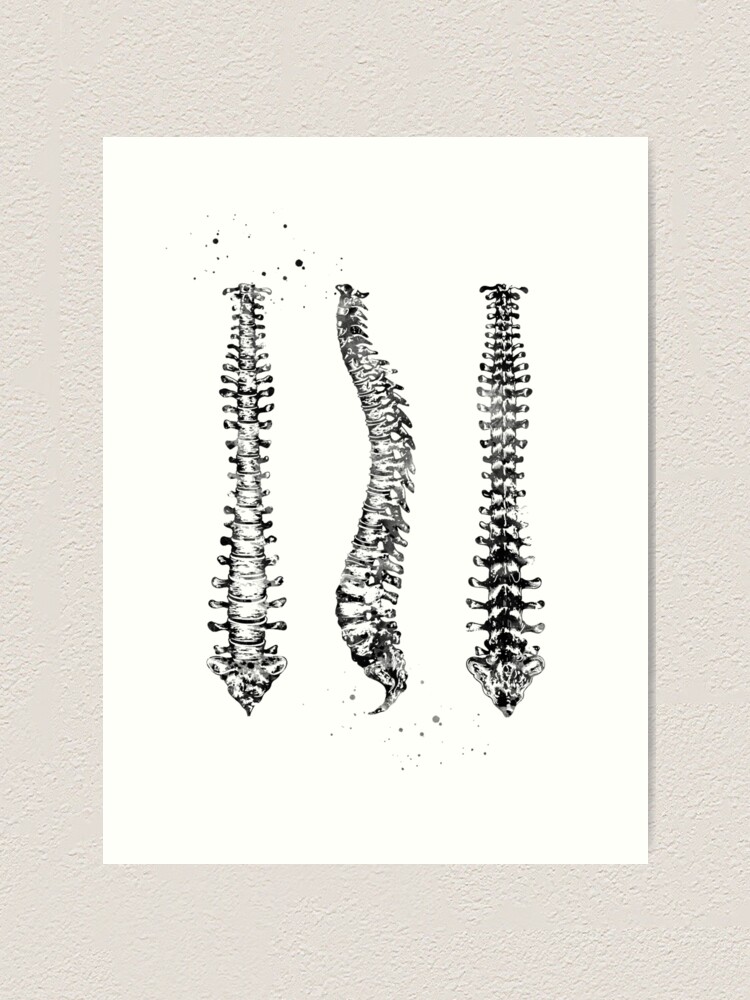The image displays a rectangular artwork in black and white, mounted on an off-white, stucco-textured wall. The artwork, set against a white background, features three intricate drawings of spines. Each spine is rendered with an inky, blotched style reminiscent of a fingerprint. The left and right spines are depicted from a top-down view, showcasing central long bone structures with protruding paddle-like bones on either side, and a small, inverted triangular shape beneath. The central spine is shown in a profile view, with a distinct curvature and similarly detailed bones. This artistic composition combines varying shades of ink, creating a visually striking contrast between the lighter and darker elements, further emphasizing the anatomical details.